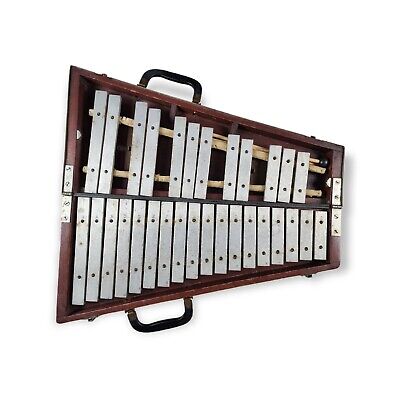This top-down photograph showcases a glockenspiel encased in a distinctive, dark mahogany-colored wooden case. The instrument features small, silvery metal bars arranged in a pattern similar to a piano keyboard, with a solid row of bars below and grouped bars above (2, 2, 3, 2, 3) akin to the black keys on a piano. The wooden case, with its sideways trapezoid shape, is open, revealing the interior components. Some bars are missing, exposing the wood underneath with empty areas beneath, adding to the instrument's charm. The open case displays two black handles on both the top and bottom, and four hinges on either side secured with silver screws, allowing the case to fold. Additionally, two long, light wooden bars, possibly mallets, are visible behind the upper keys, hinting at how the instrument is played. The varying lengths and sizes of the keys are arranged such that the smallest produce the highest notes and the largest produce the lowest.